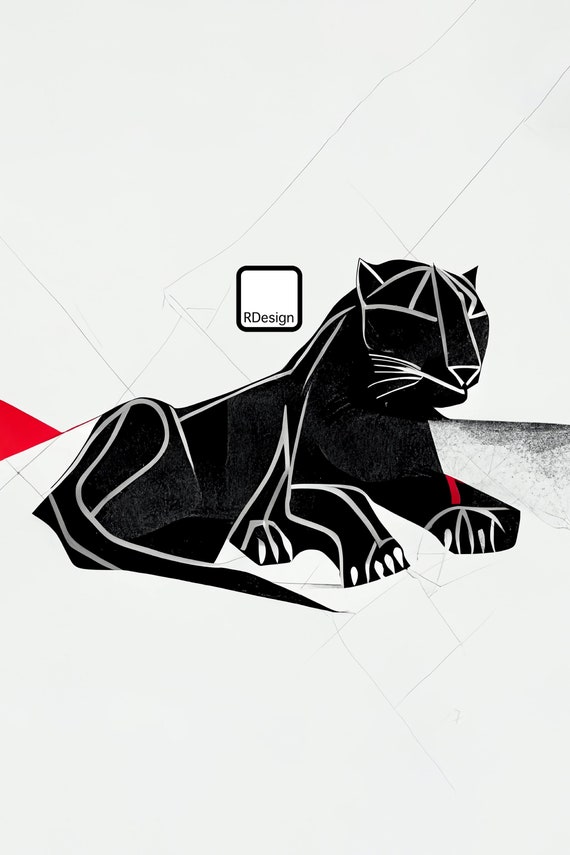The image features an abstract sketch of a cat, resembling a lion or a jaguar, composed of predominantly straight silver-colored lines with some curved parts, especially around the legs. The cat is oriented towards the right, boasting distinct characteristics such as a lack of eyes, a triangle-shaped nose, thin whiskers, and a sharp, pointy ear. Its tail, with a pointed end, curves down and back towards the front of the cat. The cat's front right paw is highlighted with a red stripe, and its claws are depicted as white, teardrop shapes that turn up and down. The background is light gray with black diagonal stripes creating a textured wall. Positioned above the cat, there is a square with rounded edges featuring a black trim and white background, displaying the text "R Design" in black letters. Additionally, a small red triangle connected to a line appears on the far left side, providing a subtle accent to the composition. The entire piece uses abstract shapes and lines to illustrate the cat, creating a visually striking, modern design.